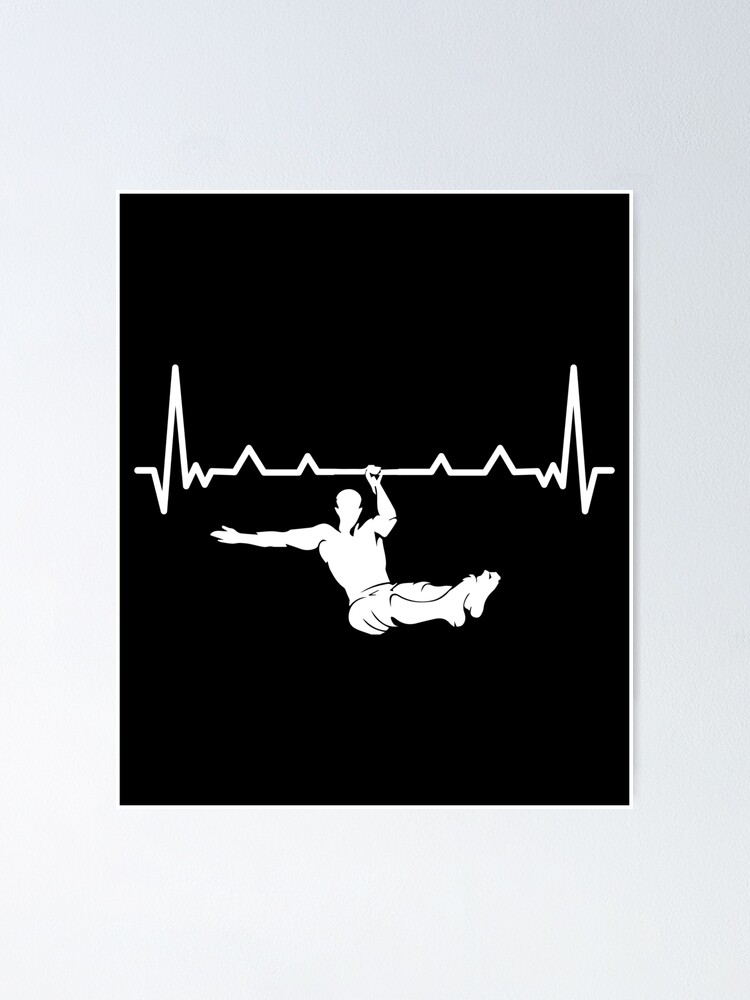The illustration showcases a minimalistic, two-toned design featuring a white silhouette of an athlete performing a calisthenics exercise against a stark black background. The athlete, shirtless and wearing shorts, is depicted hanging from an EKG heartbeat graph with his left hand, while his body is engaged in a leg lift. His right arm extends outward at a 90-degree angle, emphasizing his muscular form and athletic prowess. The graph, a spiky wave pattern symbolizing a healthy heartbeat, stretches horizontally across the image, with noticeable peaks on the left and right sides and smaller peaks in between. The entire scene, including the white figure and graph, contrasts sharply with the black backdrop, which occupies most of the space. This art piece is printed on paper with a white border and is taped to a white wall, further accentuating the minimalistic aesthetic.